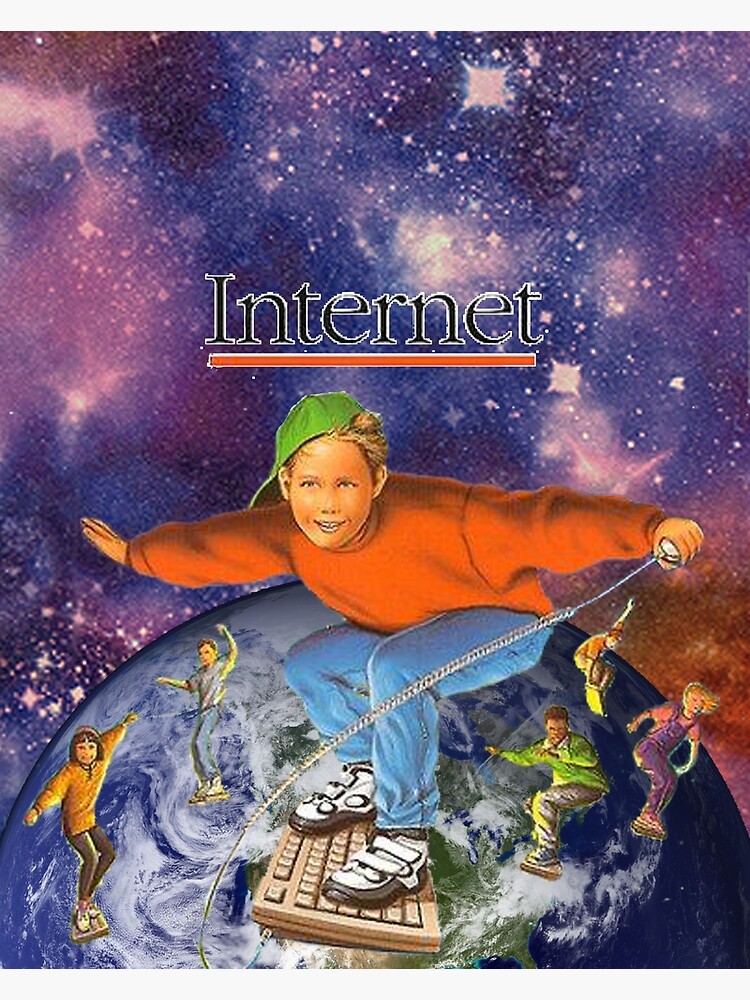The image is a stylized, cartoonish poster likely from the 1980s, aimed at advertising the internet to children. It features a young white boy around 13 or 14 years old, prominently in the foreground. He’s wearing a green baseball cap, a red sweatshirt, blue jeans, and black and white sneakers, and he's smiling as if surfing on a wave. The boy is standing on a keyboard as if it were a surfboard and holding a wired mouse in his left hand. In the background, a celestial field with a purple and lavender starburst sky frames about 60-70% of the Earth. Other children, similarly dressed, are also depicted standing on keyboards in various surfing poses, emphasizing the theme of "surfing the internet." Above the boy's head, the word "INTERNET" appears in bold black letters with an orange underline, anchoring the central theme of the poster.